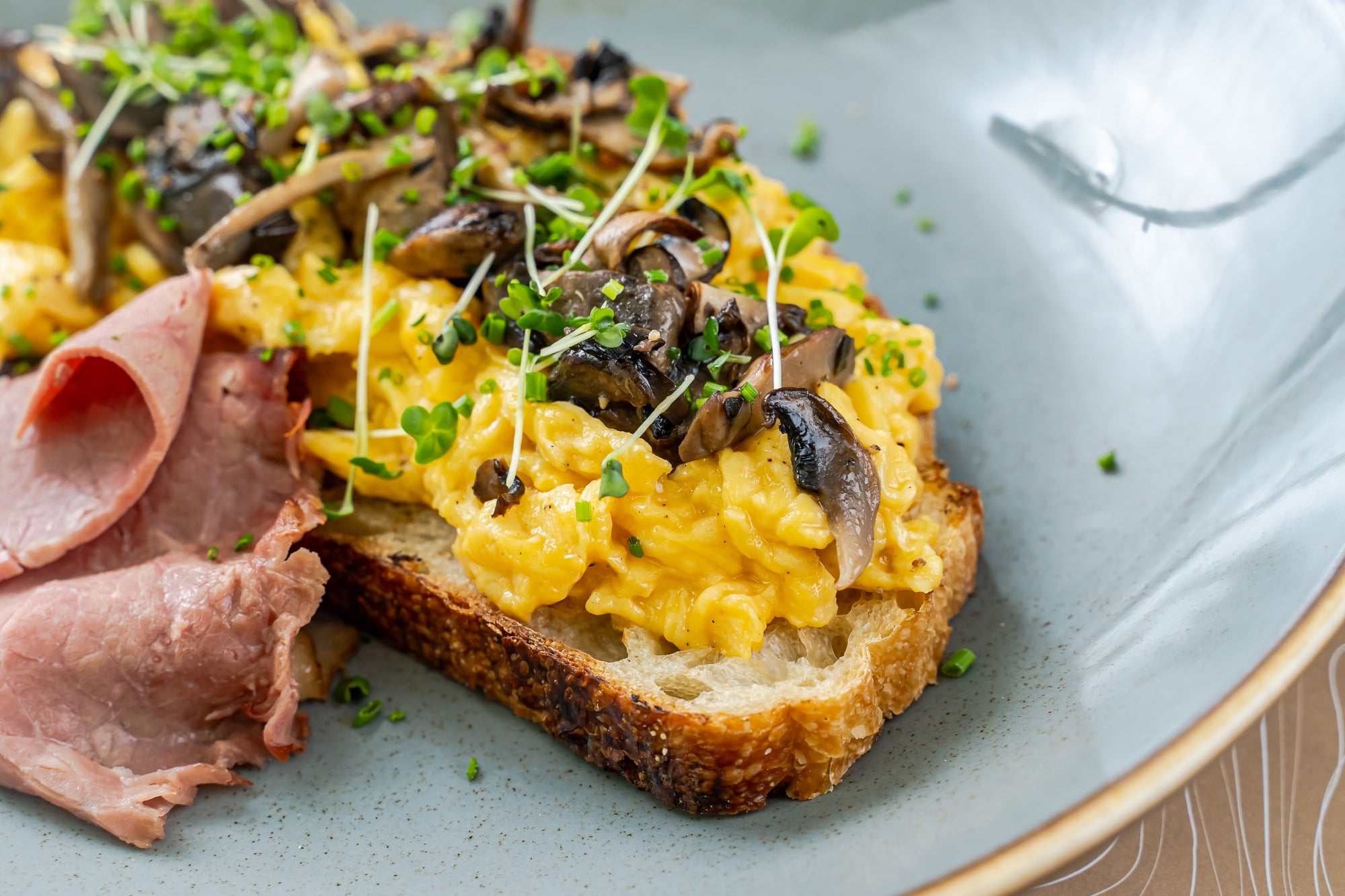In this close-up photograph of a hearty meal, a light blue ceramic plate adorned with subtle white accents occupies most of the frame, though its edges extend beyond the image. The plate is set on a brown surface with swirling white lines, possibly a tablecloth, visible in the bottom right-hand corner. On the plate, a rectangular slice of toasted bread with a dark brown crust and light brown center lies flat, its top edge arched. The toast is generously topped with dark yellow scrambled eggs, several browned mushrooms, a sprinkling of white Parmesan cheese, and scattered dark green leaves, potentially tiny sprigs of onion. To the bottom left of the toast, slightly off the image, is a pile of thinly sliced, dark pink ham, which curls up in layers. The composition and delicious overlay of ingredients suggest a filling and visually appealing dish.